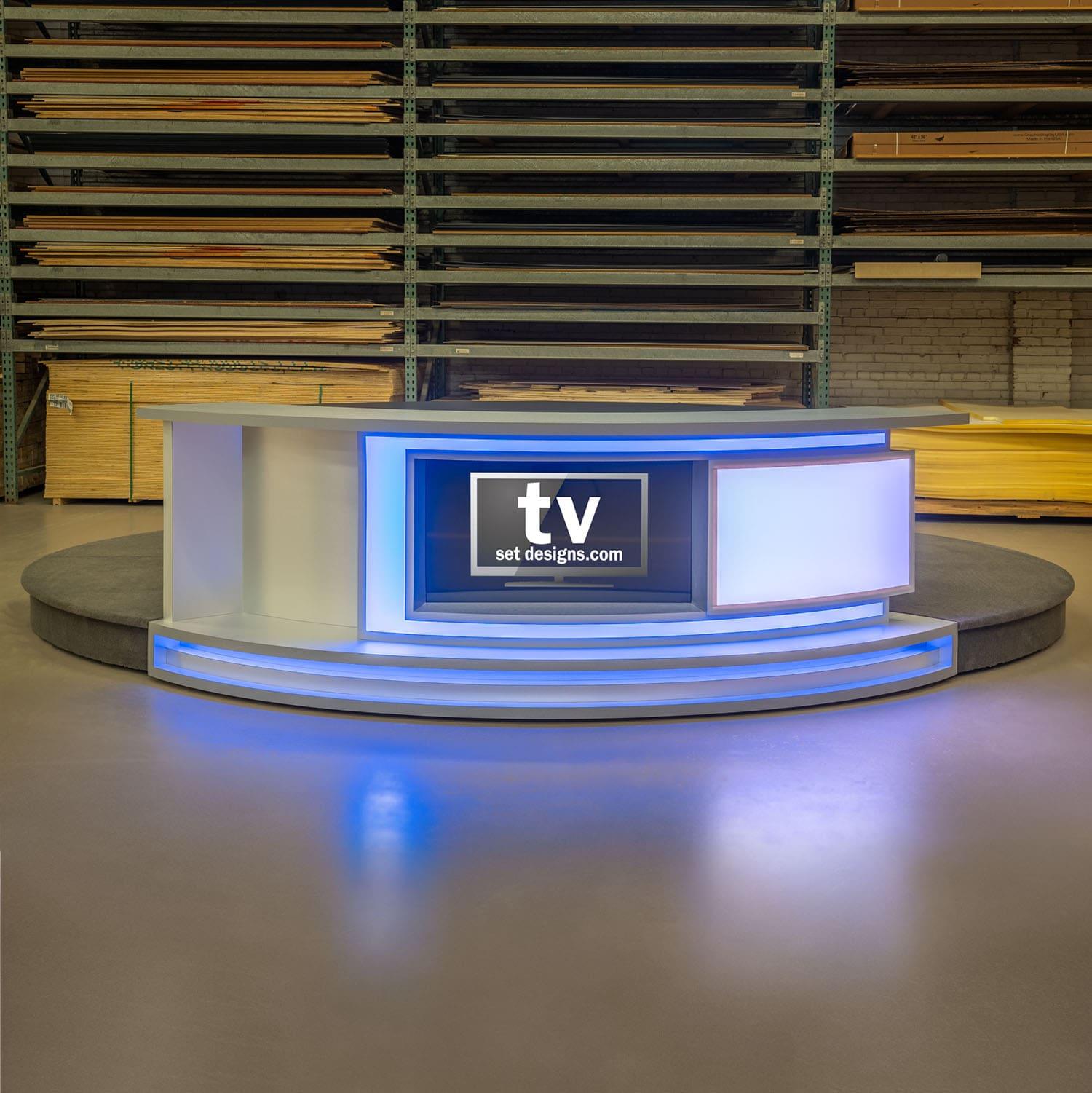This image is a detailed digital rendering showcasing a set design option, likely targeted at TV stations. The scene is set in a space resembling a hardware store or warehouse, indicated by the exposed cream-colored brick wall and greenish metal shelves stacked with long, thin pieces of plywood, reminiscent of those found at Home Depot. In the foreground, a round platform adorned with gray carpeting supports a curved desk, designed to seat the host elevated above everyone else. The desk, in a light gray or white finish, seamlessly follows the curve of the platform. Prominently displayed at the front of the desk is a screen within a TV frame, displaying the website "tvsetdesigns.com," which appears to be an advertisement for the business specializing in TV set designs. The desk is accented with blue lights, creating a subtle reflection on the smooth, concrete floor, adding a modern, polished feel to the setup.